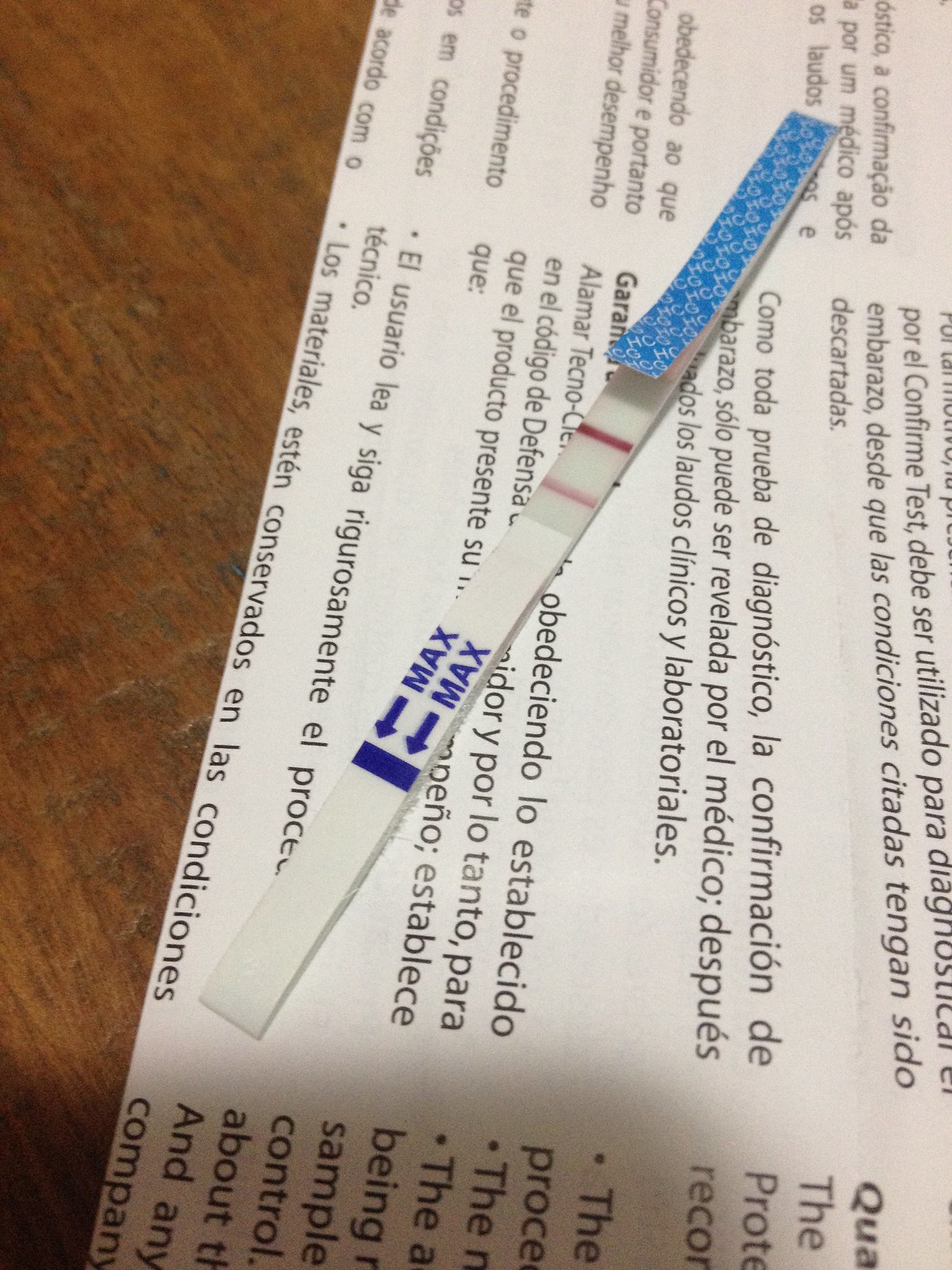This image is a detailed color snapshot of a medical diagnostic test strip, which is notably longer and thinner than a typical diabetes test strip, measuring approximately the length of a pencil. The strip is positioned on a piece of white paper featuring black printed text in Spanish, lying on a brown wooden surface, likely a table top. The table's surface shows visible nicks, scratches, and divots, suggesting regular use.

The paper, which appears folded and oriented sideways, requires one to rotate the image 90 degrees to the left to read the text correctly. Although the text is primarily in Spanish, a small portion at the bottom reveals an English section containing partially visible words such as "quality," "protective," and "process," indicating instructions related to the use of the test strip.

The test strip itself is white, with its upper portion displaying a blue and white patterned section, reminiscent of ornately designed paper. This section has two red lines, similar to pregnancy test indicators but differing in color intensity. Below this, the strip has a bright white area marked twice with the word "MAX" in blue letters, accompanied by thick blue arrows pointing towards a blue bar, suggesting a maximum fill level for dipping.

The obscured Spanish text on the paper includes phrases like "como toda prueba de diagnostico," "la confirmacion de," and "solo puede ser revelado por el medico," which translate to diagnostic test instructions and the need for professional interpretation of results. Other partially visible phrases hint at clinical and laboratory context, possibly indicating the strip’s use in drug testing or other medical diagnostics.